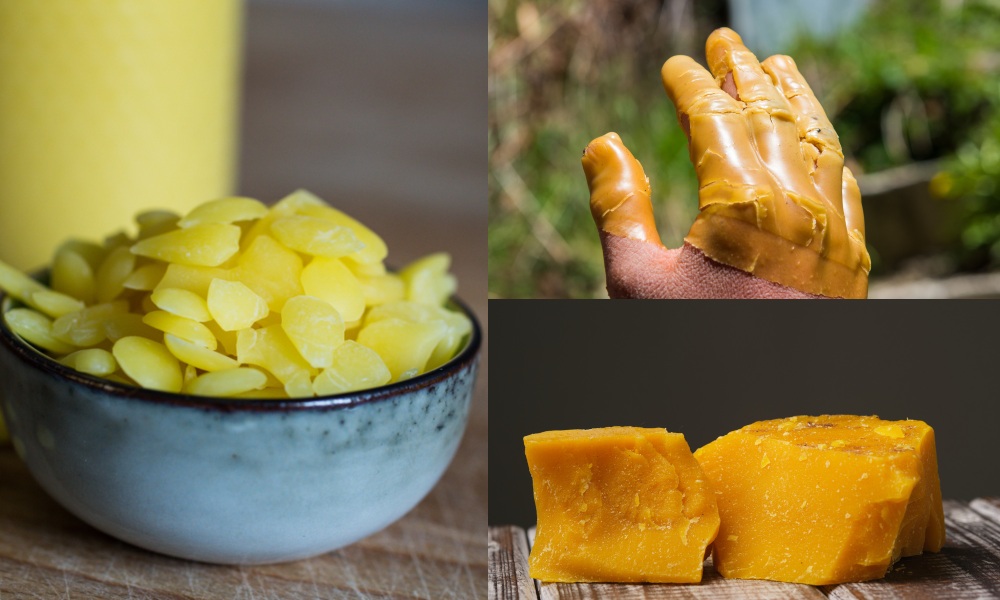The image is divided into three sections: a large photo on the left and two smaller photos on the right presented in a horizontal layout. The left side features a blue ceramic bowl filled to the brim with small yellow, wax-like pieces resembling round disks. The top right section shows a hand that appears to have been dipped in and is now covered with orange wax up to the thumb joint, framed by a blurry green background. Below this, the bottom right section displays a block of orange wax, reminiscent of cheddar cheese, placed on a wooden surface against a black background. This cohesive composition highlights the textures and colors of the wax in different forms and stages.